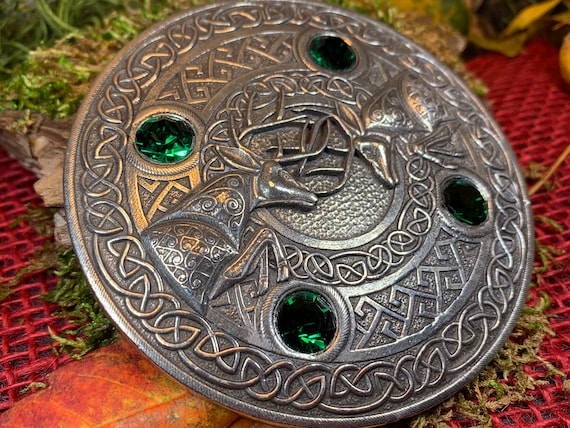This photograph captures a detailed, close-up view of an ancient shield, which dominates the frame with its round, bronze-colored, dark metal surface. At the center of the shield, two male bucks, poised in combat with their antlers locked, are intricately etched into the metal. This central motif is surrounded by geometric patterns that resemble Irish or Scottish designs, lending an ornate and historical feel to the artifact. Adding further to its richness, four deep green stones, possibly emeralds, are inlaid evenly across the surface. In the background, some red crisscrossing fabric or a net is visible, alongside orange leaves or plant matter, hinting at a natural or outdoor setting. The precise scale of the shield is unclear, but it sits prominently within the image, suggesting its significance and craftsmanship.